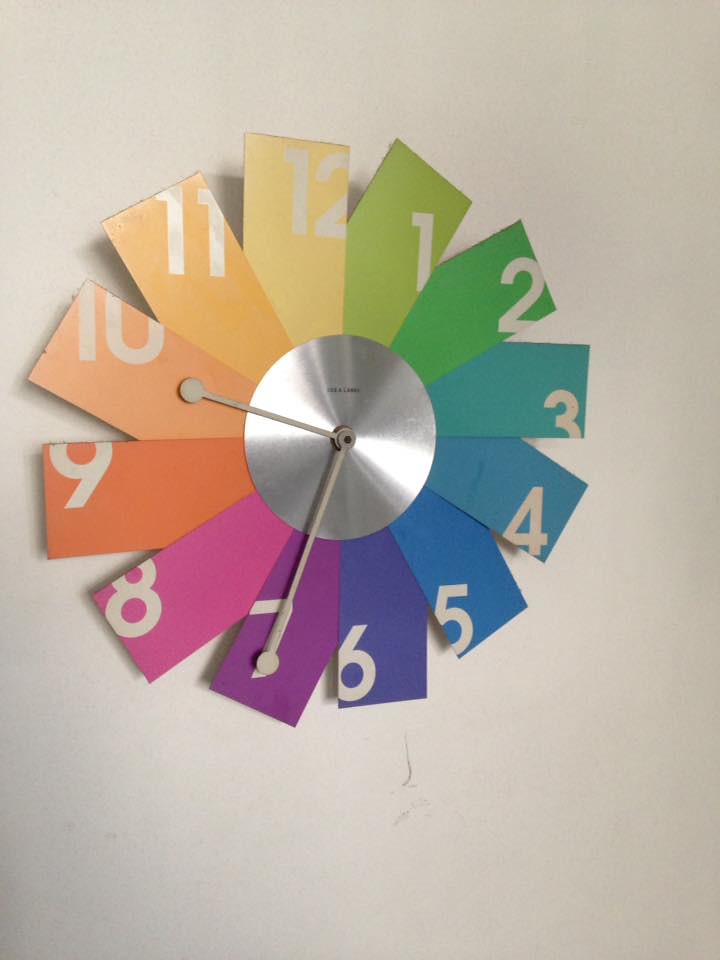The image displays a distinctive, colorful clock hanging on a smooth, white drywall. This handmade clock, seemingly crafted from reclaimed materials, features a central metallic disc resembling the reflective side of a compact disc. Highlighted on the top left and lower bottom, the silver-toned center is encircled by two plastic hands with small white dots at the tips. The hour hand points to 10, while the minute hand points towards the 7. Surrounding the central disc are rectangular paint swatches, arranged in a continuous rainbow spiral with pastel shades ranging from warm greens to mint greens, light blues to various shades of blue, purples, pinks, oranges, and yellows. Each color swatch bears white numbered markings from 1 through 12, some partially cut off at the edges. This artistic clock notably lacks minute dashes, contributing to its unique aesthetic.